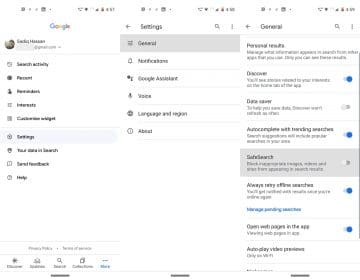This rectangular image features a very blurry and small screenshot. At the top of the screen, faint and indistinguishable small icons are visible, appearing merely as gray squares and dots. Below these icons, in the upper left corner, the word "Google" is faintly recognizable by its colors, although the letters themselves are hard to discern. 

To the right of "Google," the word "Settings" appears in black text, accompanied by a left-pointing arrow. Adjacent to this, on the left side of the arrow, there is a general arrow icon also pointing left. Further right, there is a search magnifying glass icon.

Below the word "Google," on the left side of the screen, a round circle contains a name, with the first letter "S" and the first letter of the second name being "H". Another round circle to the left displays a headshot, likely a black and white image of a person's head.

Vertically aligned beneath this, the text reads "Search activity," followed by a series of other words, which are partially discernible as "personal," "interest," "settings," "search," and "help." 

To the right of these vertically listed words, the terms "settings," "notifications," "language," and others appear, which are difficult to distinguish due to the blurriness of the image.